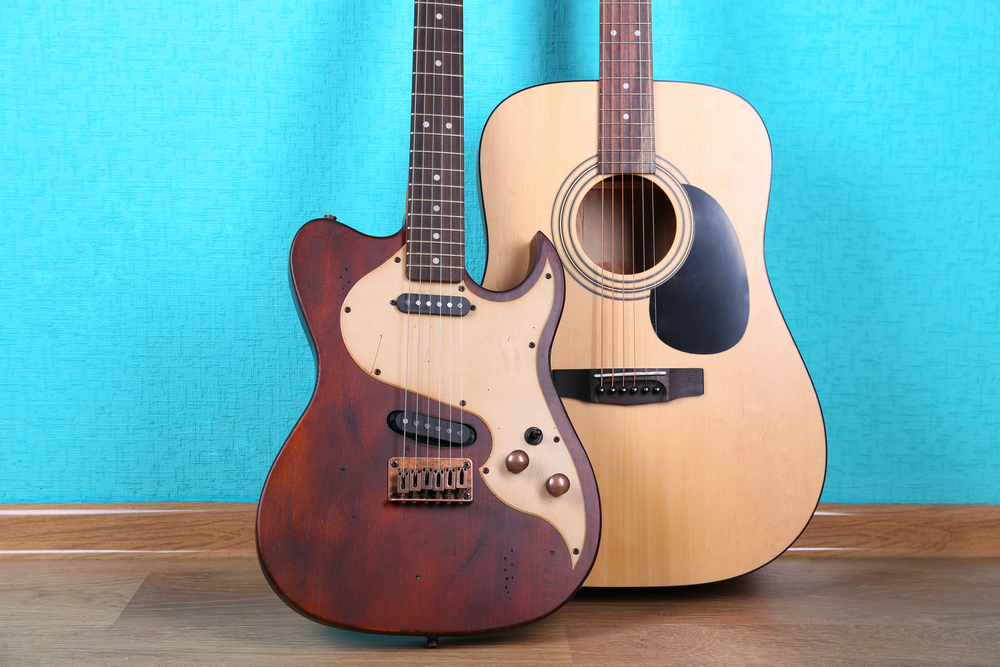In the image, two distinct guitars are leaning against a bright blue wall with a wooden baseboard. Both guitars rest on a wooden floor. The guitar in the foreground, positioned on the left, is an electric guitar with a body crafted from dark wood with a flame-like light wood section on the right side. It features six metal strings and a port or jack for plugging in an aux cable. The neck of the electric guitar is made from dark wood. Just behind this guitar, partially obscured, is an acoustic guitar. This acoustic guitar has a light wood body with a pronounced black circle around the sound hole, which is accompanied by a black slap panel. The acoustic guitar's neck is also dark wood but slightly lighter than that of the electric guitar. Both guitars' six strings are arranged differently – nylon strings with varied colors on the acoustic guitar. The scene is set against a vibrant blue wall and the instruments rest on a wooden floor.